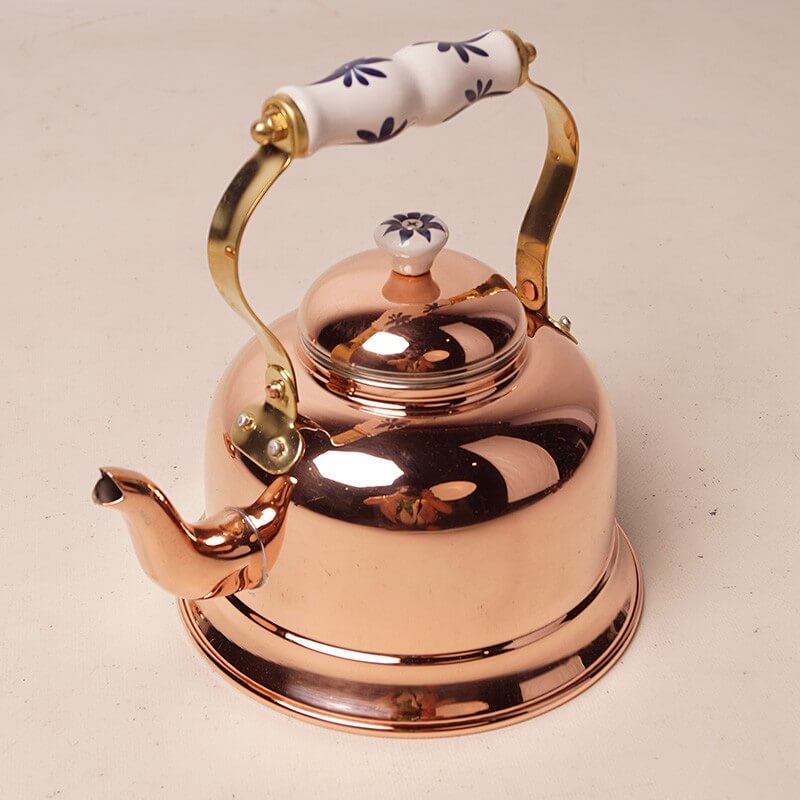This image depicts an ornate, vintage copper teapot with a lustrous, rose-gold hue, positioned on a pinkish-beige background. The teapot, exceedingly reflective, mirrors its surroundings, including the photographer, indicating its polished, shiny surface. The teapot's body flares slightly at the base, culminating in a dome-shaped lid, topped by a small, white ceramic handle adorned with blue floral patterns. The main handle, golden in color, could be brass, and arcs gracefully to join a flat upper section also fashioned with white ceramic, decorated with blue flowers for grip. Additionally, the spout, located on the left, features a snake-like curve and a carved notch at the mouth, contributing to the teapot's elegant and intricate design.